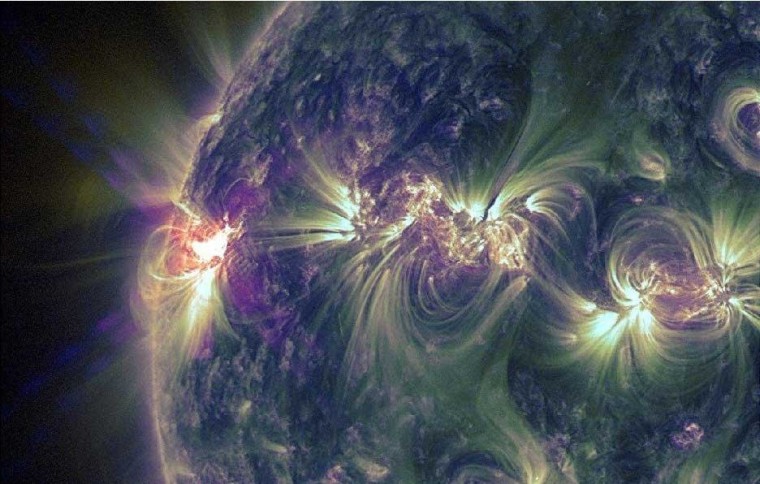The image depicts a close-up, likely satellite-taken, infrared photograph of the Sun or a similarly large celestial body. Dominating the right side of the image, the celestial body exhibits a darkened, bluish-green mass. Along its curved left edge, the contrast is stark against the blackness of space. A striking feature of the photo is a band of bright solar flares or possibly sunspots, arrayed across the middle of the Sun. These flares or hot spots emit radiant green and purple colors, with tendril-like extensions swirling outward, almost appearing as waves of radiation or heat. There are three or four prominently visible flares, accompanied by swirling green gas-like matter extending above them. The rest of the Sun showcases a mix of bluish-beige hues, further accentuated by occasional orange light from the flares.